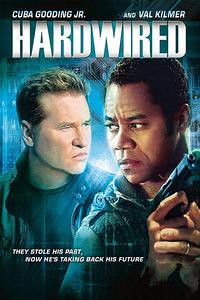The movie poster for "Hardwired" prominently features Cuba Gooding Jr. and Val Kilmer against a dramatic backdrop. Cuba Gooding Jr., positioned at the right center, holds a gun with a clenched, tense expression while looking off to his right. Val Kilmer is placed to the left center, also appearing tense, with a furrowed brow, gazing to his left. The top of the poster displays their names in small white print, with "Cuba Gooding Jr." on the left and "Val Kilmer" on the right. Below their names, the movie title "Hardwired" is boldly printed in large white letters. The lower left corner features a smaller caption in white, stating, "They stole his past. Now he's taking back his future." The visual theme of the poster predominantly uses shades of blue, with natural skin tones and hair colors contrasting against the moody background; Cuba's black hair and Val's blondish-brown hair are prominently visible. The composition and digital creation of the image emphasize a high-stakes narrative, capturing the intensity and tension of the film.